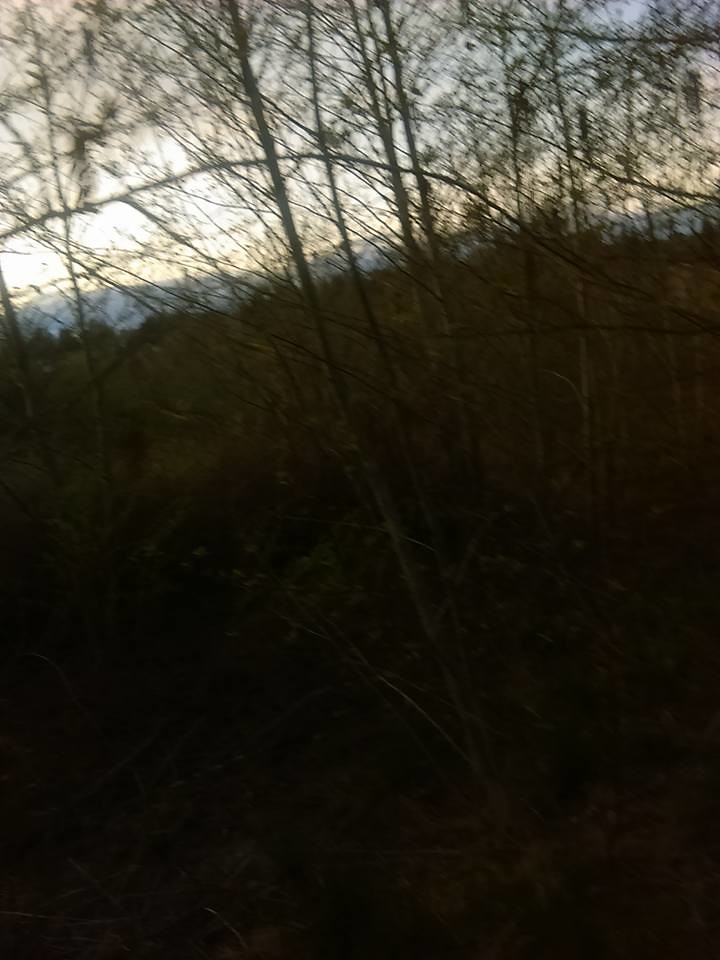A dense forest appears in this image, shrouded in dim light and filled with numerous tall trees. The forest floor is a chaotic tapestry of fallen trees, branches, and twigs, intermixed with dark brown brush. Some of the trees in the foreground are leafless, suggesting it might be fall. Through the nearby trees, which obscure parts of the view, the distant horizon reveals sunlight bathing the tops of majestic mountains. The dense forest extends endlessly towards the horizon, a wild expanse of trees and brush stretching as far as the eye can see.